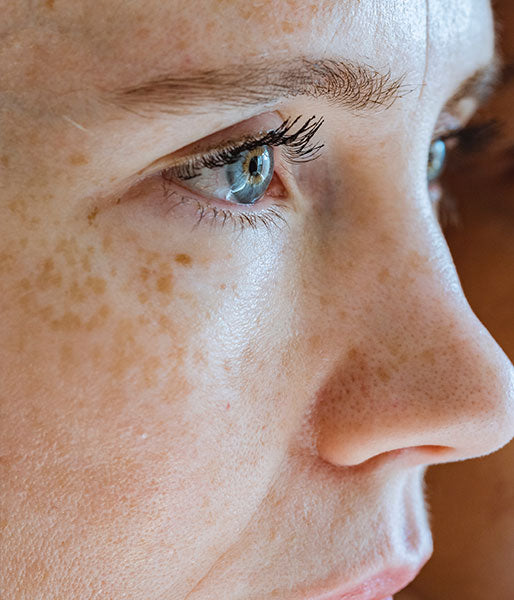This extremely close-up photograph captures the upper half of a Caucasian woman's face, focusing from just above her upper lip to about an inch above her eyebrows. The side profile highlights her pale skin adorned with freckles scattered mainly under her eye, along her nose, and on her cheek. Her striking blue eyes, framed by black mascara-coated eyelashes and brown eyebrows, stand out prominently. The image also reveals the texture of her skin, including visible pores on her nose and a hint of fine fuzz above her natural-shaded lips. A portion of the background, beyond the right side of her face, is a muted brown, adding depth to the detailed and intimate portrait.